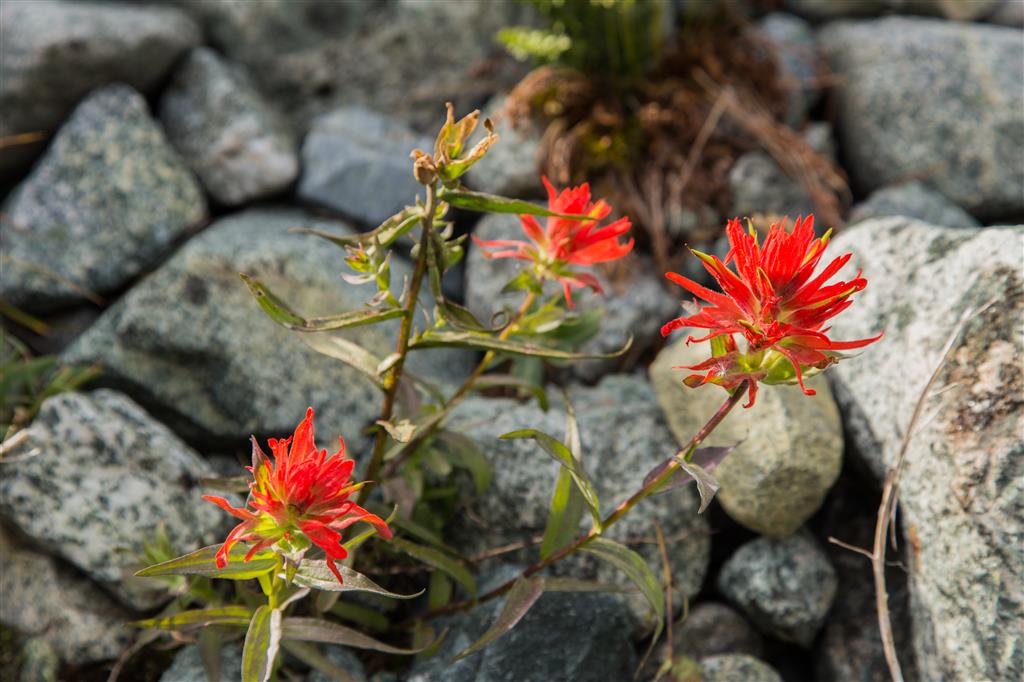This outdoor scene captures a vibrant plant growing amongst an array of large gray rocks speckled with black. Radiating in the daylight, the plant features greenish-brown stems adorned with narrow, pointy green leaves. Atop these stems, there are three vivid red blooms, each flower boasting numerous long, narrow petals with subtle yellowish tips. Additionally, there's a dried, dead flower near the upper middle of the image, slightly off to the left. The backdrop includes patches of dead vegetation, visible grass, and a prominent dead stick on the right side. The sunlight accentuates the lively colors of the flowers contrasted against the muted tones of the rocky background.